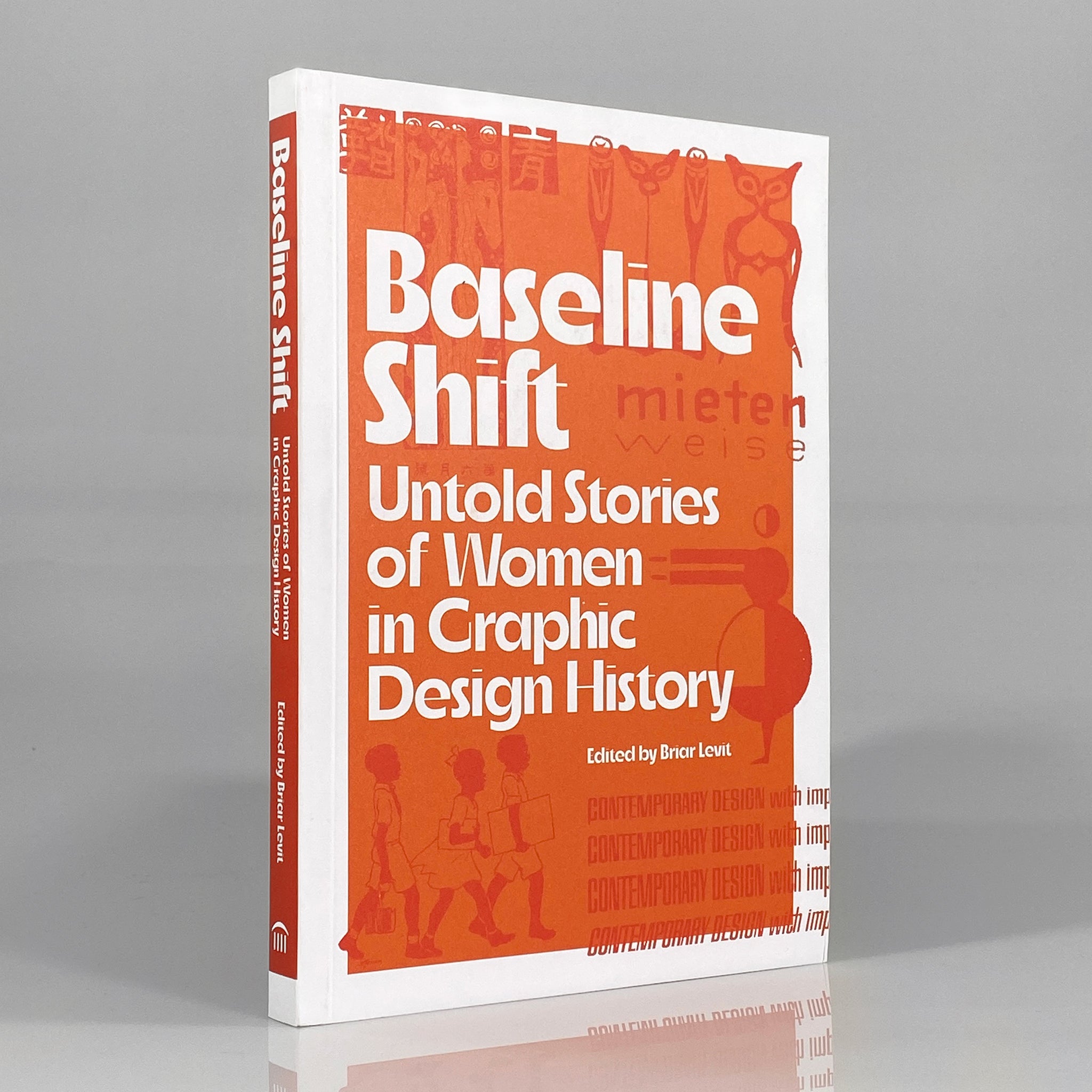The image is a product photo of a book titled "Baseline Shift: Untold Stories of Women in Graphic Design History," edited by Briar Levitt. The book stands upright on a reflective, flat gray surface with a matching gray background. The cover is predominantly orange, enclosed by a white border that also frames the spine. The title is prominently displayed in large, white, funky-looking text, with the subtitle and editor's name in smaller white text beneath it. The orange cover is adorned with darker orange, almost red designs, which include diverse elements such as indigenous or Mayan-like artwork at the top, lab equipment on the right, Chinese figures, and silhouettes of three young children. Additionally, there's an image of a stick figure woman in an apron and some slightly obscure text in orange on the cover. The overall design features intricate, thematic illustrations that enhance the book's striking presentation.